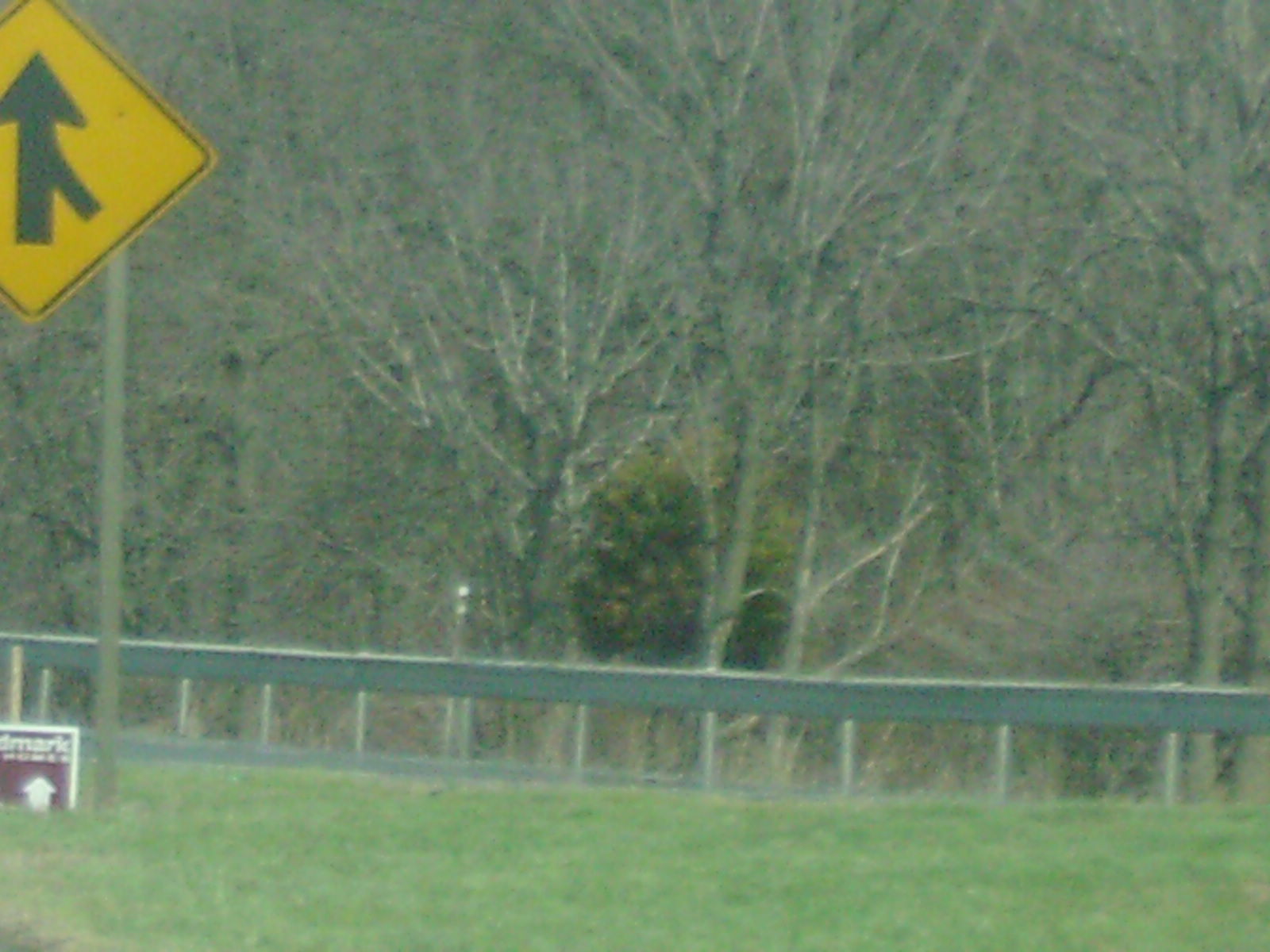This outdoor daytime image captures a scenic field of grass that stretches across the bottom middle of the picture. On the left side of the image, prominently featured, is a large wooden post that extends vertically. Attached to this post, at the middle height, is a yellow diamond-shaped sign with a black upward-pointing arrow. Slightly below and to the left, there is a smaller purple sign partially visible, displaying the letters "DMARC" on a reddish background along with a white upward-pointing arrow. Beyond the grassy field, a short metal railing with a horizontal gray bar runs across, acting as a barrier before reaching the wooded area in the background. The majority of the trees in this wooded area are devoid of leaves, suggesting a season like fall, winter, or early spring. Notably, one short tree stands out with its dark green and yellowish leaves, contrasting against the otherwise barren backdrop.